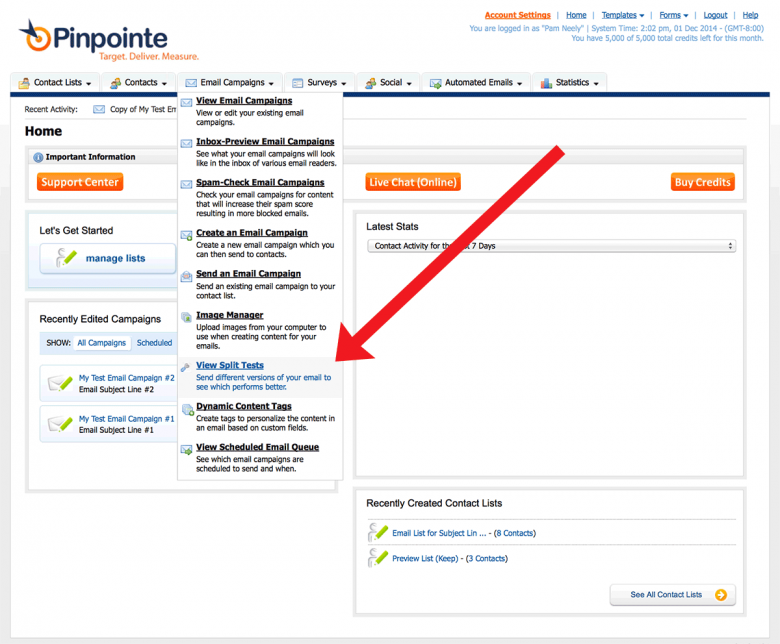This image, sourced from the "Pinpoint Target, Deliver, and Measure" website, showcases a detailed interface of an email marketing platform. At the heart of the image is a prominent red arrow that diagonally traverses the screen, directing attention to a specific feature labeled "View Split Test." This feature, described as a tool for sending different versions of an email to evaluate performance, is positioned in a middle-left column on the screen.

The interface's top navigation bar displays several sections: "Contacts," "Email Campaigns" (the current open section), "Surveys," "Social," "Automated Emails," and "Statistics." Above this, the uppermost menu features options in orange and blue, including "Account Settings," "Home," "Templates," "Forms," "Logout," and "Help."

Further down, within the "Email Campaign" section, users can access multiple functionalities such as "View Email Campaigns," "Inbox Preview Email Campaigns," "Spam Check Email Campaigns," "Create an Email Campaign," "Send an Email Campaign," "Image Manager," "View Split Test" (highlighted in blue), "Dynamic Content," and "View Scheduled Email." Each feature is clearly listed, guiding users through the various tools available for managing and optimizing email campaigns.